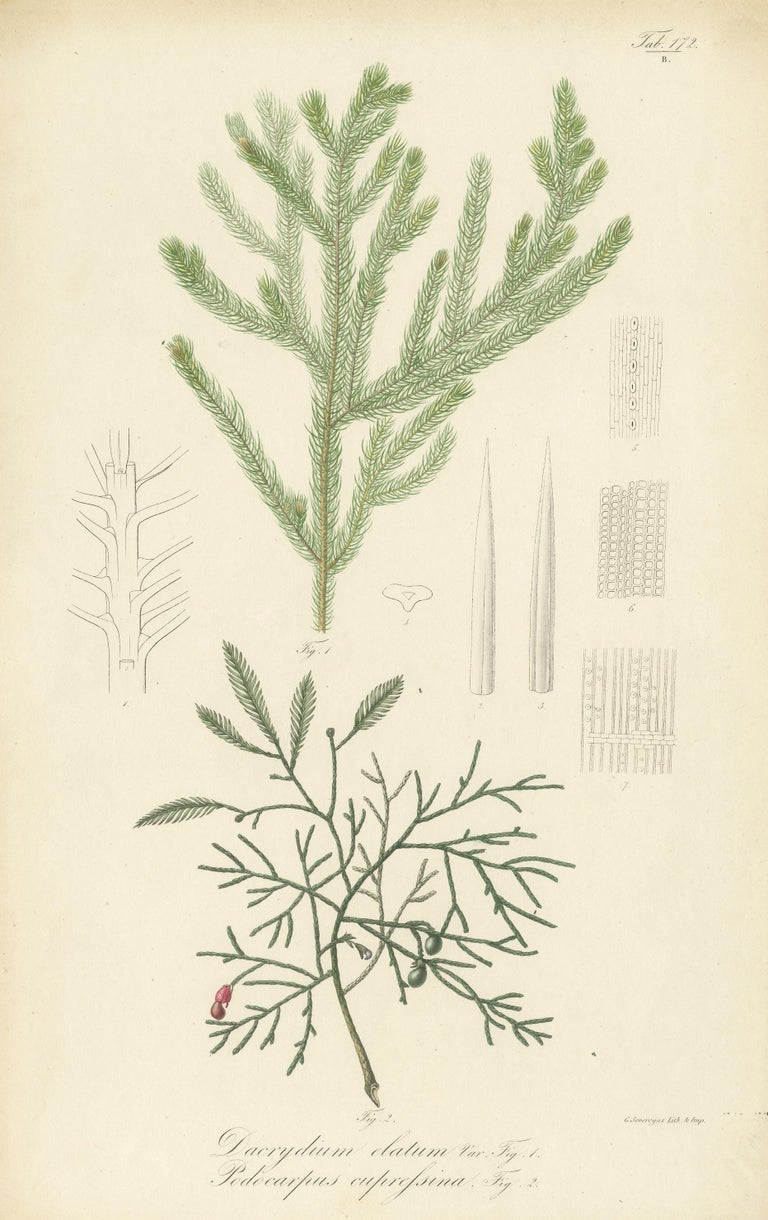The image depicts a portrait-style botanical illustration on aged, yellowed paper, which darkens towards the edges. At the top, a central brown branch features small green pine needles arranged along its length. Surrounding this main branch are black and white sketches of various other plants, including a portion of a tree trunk with branches extending from it, and a collection of lines, dots, squares, and rectangles, which may represent detailed botanical sketches or annotations. Below this, there is another plant with bare branches for the most part, except for the top portion where small green leaves and two prominent red berries are visible. The bottom of the illustration features thin cursive writing which reads "Daracidium daelum, Pedicuripus euphrycina," along with labels "fig 1" and "fig 2." Overall, the illustration presents a detailed study of different plant species with a focus on the contrast between the brown and green shades of the branches and leaves.